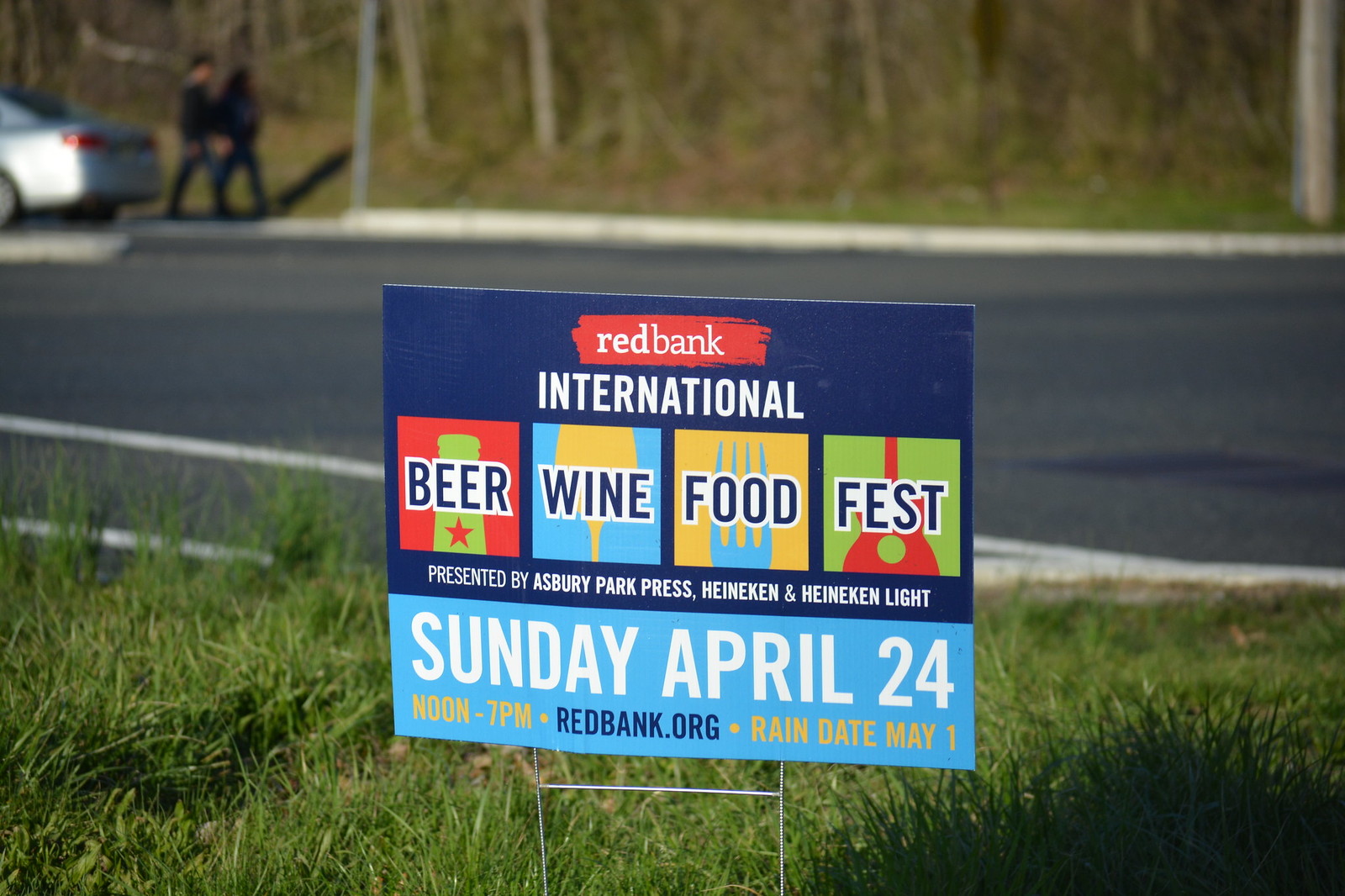The image captures a small, wire-framed yard sign placed in a patch of long green grass along the side of a two-lane road. The sign, which appears to advertise an event, features a dark blue background at the top fading to light blue at the bottom, with a narrow red band at the top that reads "Red Bank" in white text. Beneath this, the word "International" is written in white. The sign is divided into four colored squares, each listing a different attraction: the first square, in red, displays the word "Beer" alongside the top of a green Heineken bottle; the second square, in blue, says "Wine" with a yellow wine glass icon; the third, in yellow, reads "Food" with a blue fork illustration; and the fourth, in green, states "Fest" next to what appears to be a guitar silhouette. The sign announces the "Red Bank International Beer, Wine, Food Fest," presented by Ashbury Park Press, Heineken, and Heineken Light. The light blue section at the bottom of the sign provides event details: "Sunday, April 24, noon to 7 p.m.," with a rain date of May 1st, and the website "redbank.org."